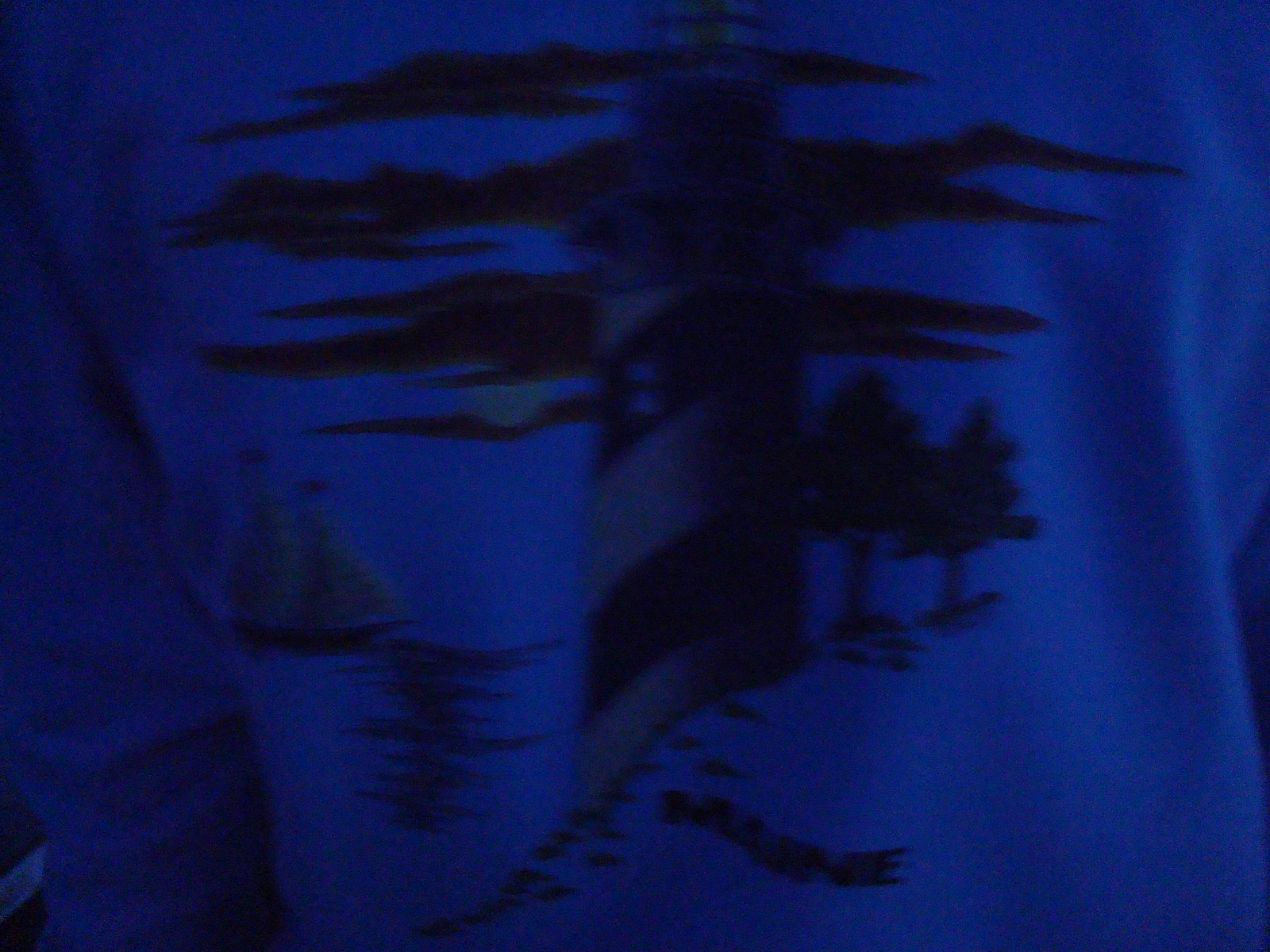In the image, there is a close-up of a dark-hued long-sleeve t-shirt with a prominent bluish filter. The shirt appears to be either light blue or white, obscured by the dark and blurry quality of the photograph. Dominating the center of the shirt's graphic is a tall lighthouse with distinctive candy cane-like diagonal stripes in alternating tan and green, or possibly white and black due to color distortion. The lighthouse stands majestically against a backdrop of black clouds, partially covering the sky. To the lighthouse's left, the design features a historic wooden sailboat navigating the ocean, which reflects the sky above. Two trees stand to the right of the lighthouse, adding a touch of land to the maritime scene. At the bottom of the shirt, the word "Maine" is boldly printed, signifying the location or inspiration of the graphic.